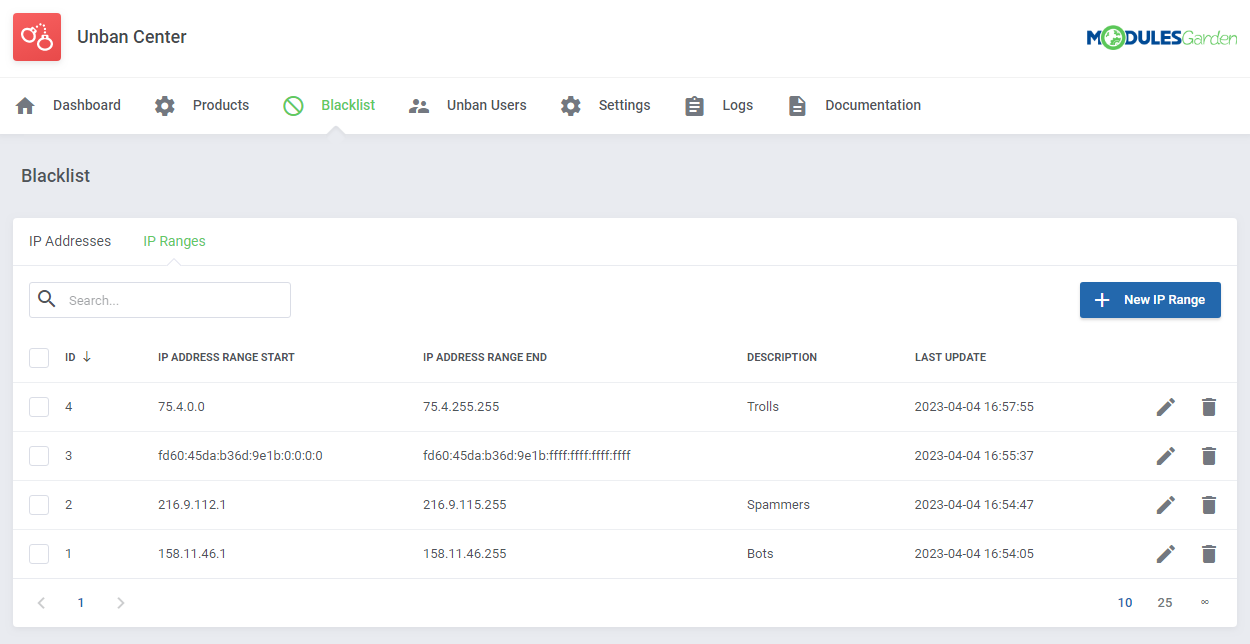This screenshot captures the user interface of the "Modules Garden" software. Dominating the upper right corner is the brand logo, which features a stylized "M" in blue. The "O" is represented by a green Earth, followed by "DULES" in all-caps blue letters. The word "Garden" is italicized with a capital "G," rendered in green font.

To the left, a red square icon with white handcuffs is labeled "Unban Center." Below this, there's a series of navigation tabs, each accompanied by an icon:
- **Dashboard:** Home icon
- **Products:** Settings gear icon
- **Blacklist:** Currently selected, highlighted in green text with a green cancel-circle icon
- **Unban Users:** Two portraits icon
- **Settings:** Gear icon
- **Logs:** Clipboard icon
- **Documentation:** Google Forms-like paper icon

In the central section, a gray header displays the text "Blacklist." Beneath this, a white page contains two tabs: "IP Addresses" and "IP Ranges," the latter being currently selected and highlighted in green.

A table-display area begins with a search bar, while a blue action button labeled "New IP Range" with a white plus sign is positioned in the top right corner. The table, which sorts data by columns, shows four results sorted by ID: 4, 3, 1, and 2. The available columns include:
- IP Address Range Start
- IP Address Range End
- Description
- Last Update

Each row ends with Edit (pencil icon) and Delete (trashcan icon) actions. The descriptions in the table include terms like "Trolls," "Blank," "Spammers," and "Bots." The "Last Update" column captures both dates and timestamps, and the IP Address Ranges consist of standard numerical dot-separated values.